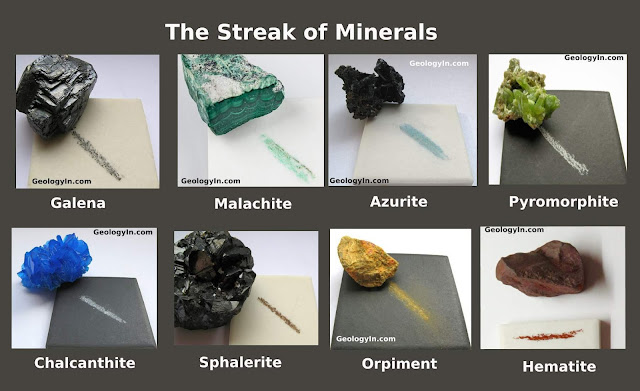This detailed photographic image, titled "The Streak of Minerals," showcases eight distinct minerals arranged on a charcoal gray background. The display is divided into two rows, each featuring four minerals. 

From left to right in the top row, the first mineral, Galena, is a dark, grayish rock resting on a cream block, creating a black streak. To its right, Malachite, a glistening teal mineral, sits on a white block and leaves a teal streak. Next is Azurite, a black, charcoal-like mineral, also on a white block, which produces a blue streak. The fourth mineral on this row is Pyromorphite, a lime-green, irregularly shaped stone on a dark grey block, which leaves a white chalk-like mark.

The bottom row begins with Chalcanthite, a bright crystal blue mineral on a black block, leaving a white streak. Next is Sphalerite, a dark gray, almost black mineral on a white block, creating a dark brown streak. Orpiment is next, a stone with orange-yellow hues on a grey block, leaving a similarly colored bronze streak. The row concludes with Hematite, a reddish-brown mineral on a white block, producing a red streak.

Each mineral is annotated with its name in white text along with the streak it leaves, serving as an instructive visual aid. Additionally, the website "geologyn.com" is mentioned in small text at the bottom of each mineral's photo.